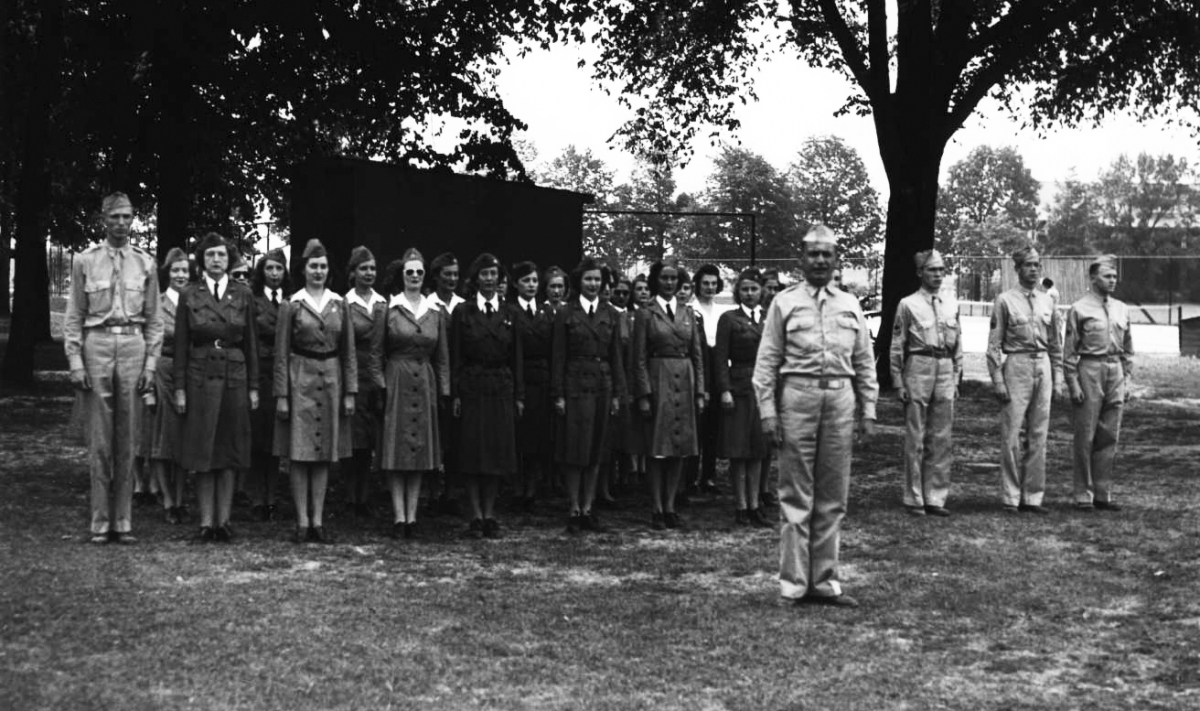This is a historical black-and-white photograph capturing an outdoor scene likely set at a training camp. The image is horizontal-rectangular, showcasing a group of uniformed individuals standing at attention. In the foreground, a man in a khaki military uniform, standing somewhat centrally but towards the right, commands attention with his hands at his sides, wearing what appears to be a navy-style hat. Surrounding him are several other men in similar khaki uniforms, positioned primarily towards the perimeter of the group.

Among them, a mix of approximately 15 to 20 women can be seen. These women are dressed in various uniforms, some in darker shades and others in medium-dark attire, potentially a formal uniform with hats, ties, or blouses paired with long skirts featuring prominent buttons. To the left side of the image, there are additional men, similarly in military attire, standing in an orderly fashion.

In the backdrop, the scene is framed by large trees and an indistinct building without any signage, suggesting an institutional setting. The sky, though rendered in grayscale, is visibly clear and light, indicating daytime. The overall composition and attire hint at a formal or ceremonial gathering, reflecting a disciplined and structured environment typical of a military installation.